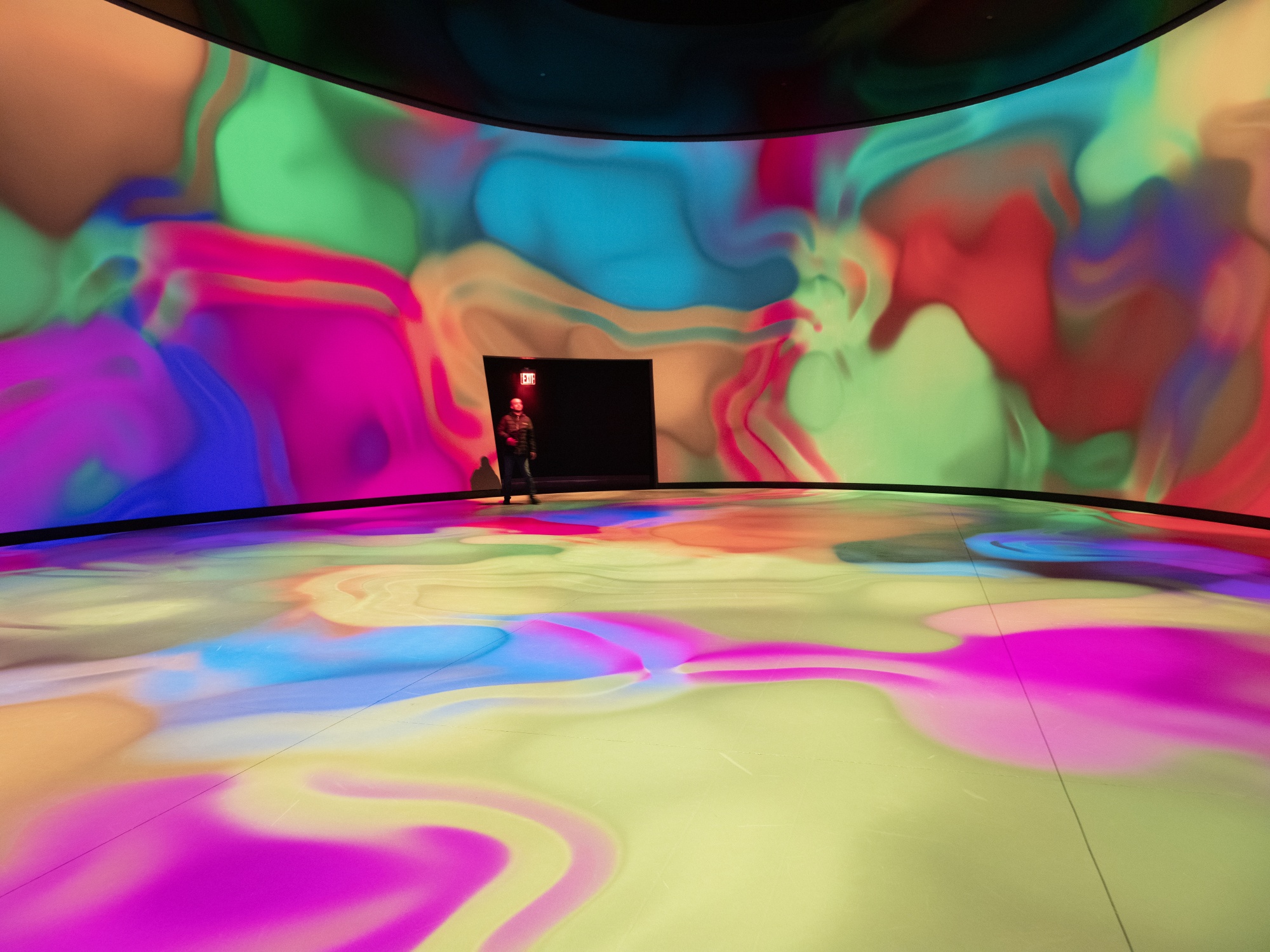This is a color photograph depicting a man on a stage, seemingly giving a talk or lecture, reminiscent of a TED Talk setting. The stage is a squarish, horizontal rectangle with a predominantly black backdrop, interrupted by a rectangular cutout that serves as an exit, marked by a blurred, illuminated exit sign. The man stands centrally in front of this opening, which is flanked by vibrant, projected patterns creating a semicircle around him. The room and stage are adorned with a spectrum of colors, including vivid hues of blue, red, lime green, purple, yellow, orange, and pastel shades of pink and blue. These colors blend into each other in wave-like patterns, giving the scene a dynamic and colorful ambiance. The beige floor also reflects an array of projected lights, forming images resembling flowers and adding to the overall vibrant atmosphere.